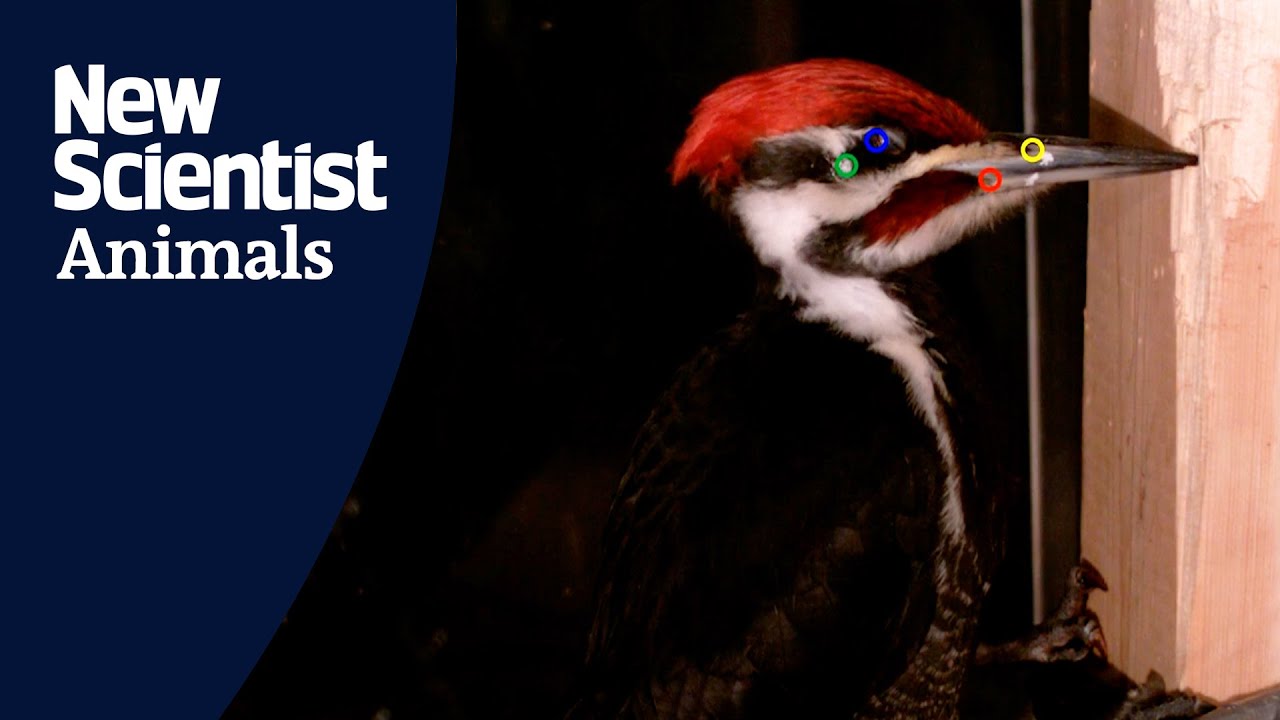This striking magazine spread features a close-up photograph of a red-headed woodpecker, prominently displayed on the right-hand side of the image. The bright red tuft on the bird’s head contrasts vividly with the intricate black and white markings that adorn its body, extending from its head down to its belly. The woodpecker’s piercing green eye is highlighted by a blue circle, while additional colored circles—green, red, and yellow—point out specific features on its head, beak, and mouth. The bird’s long beak, directed towards the right, is positioned in front of a tall wooden pole that appears to have been chipped away by the bird’s persistent pecking. The woodpecker clings to the pole with its claws. To the left of the bird, against a dark navy background, bold white lettering spells out "New Scientist Animals," adding a clean, modern aesthetic to the overall composition. This visually engaging and detailed presentation captures the vibrant essence of the woodpecker and seamlessly combines illustration elements with photographic realism.